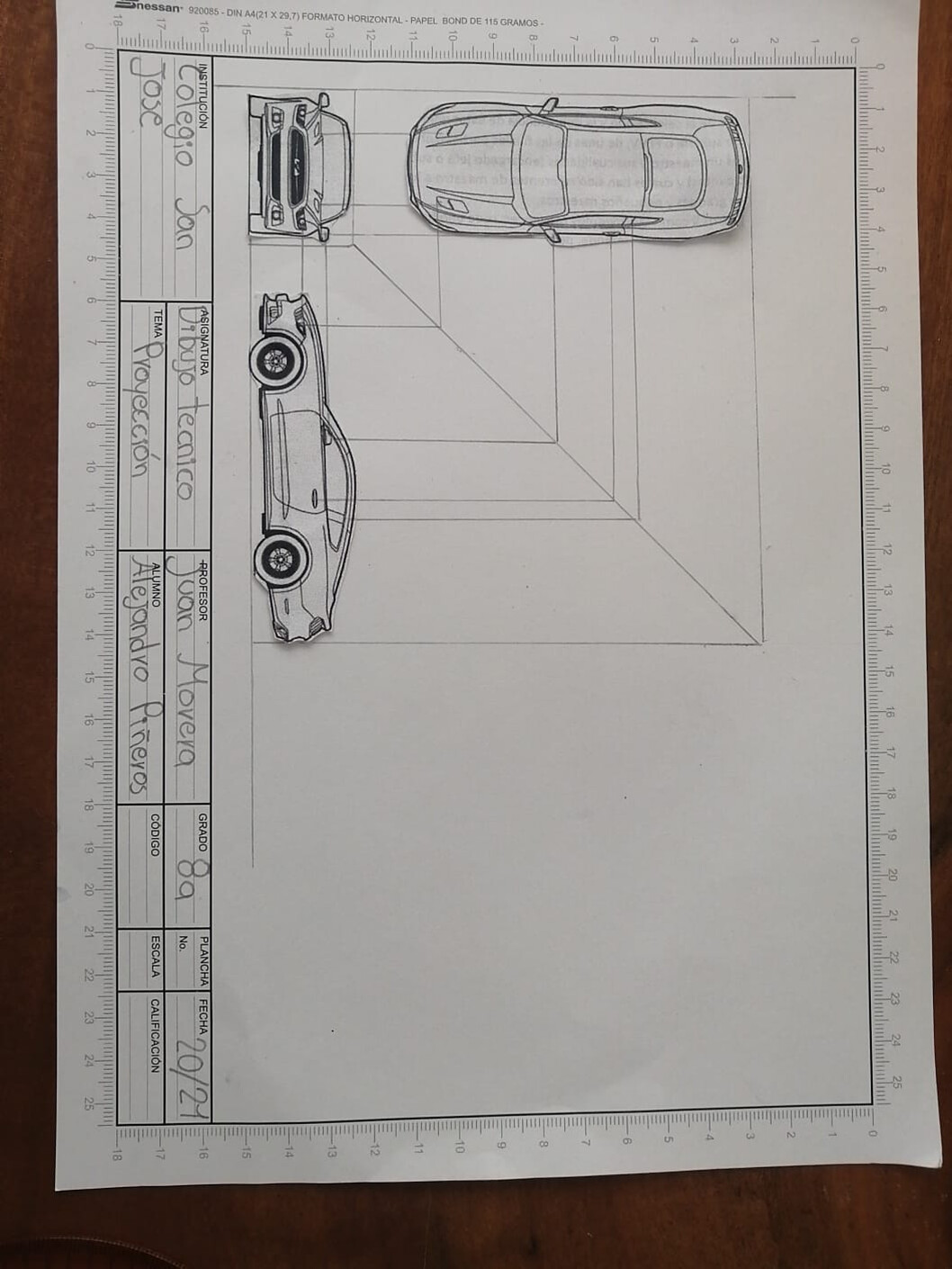The image is a detailed black and white sketch of a sleek, potentially expensive, two-door coupe car, presented on a white piece of paper oriented sideways on a black or dark wooden table. The sketch showcases three different views of the car: an overhead view with the front of the car on the left and the back on the right, a front view displaying the headlights, rearview mirrors, and grille, and a side view with visible doors and wheels. 

Around the edge of the paper, there is a rectangular ruler-like border, possibly marked in centimeters or inches, suggesting precision in the drawing. The top side, positioned to the left due to the orientation, features several labeled sections in Spanish, including:
- "Institución: Colegio San Jose" (Institution: San Jose School)
- "Asignatura: Dibujo Técnico" (Subject: Technical Drawing)
- "Tema: Proyección" (Theme: Projection)
- "Profesor: Juan Movera" (Teacher: Juan Movera)
- "Alumno: Alejandro Piñeros" (Student: Alejandro Piñeros)
- "Grado: 8a" (Grade: 8th)
- "Fecha: 20/21" (Date: 20th/21st) with some sections left unfilled.

The paper's texture and weight are described as "papel bono de ciento cincuenta gramos" (150-gram bond paper). The sketch also seems to include the word "Nissan" on the side of the car and showcases detailed measurements and annotations, indicating the educational and technical intent of the project. The artist's signature, "Colosio, San Jose," is written sideways along the edge, adding a personal touch to this meticulously crafted technical drawing.